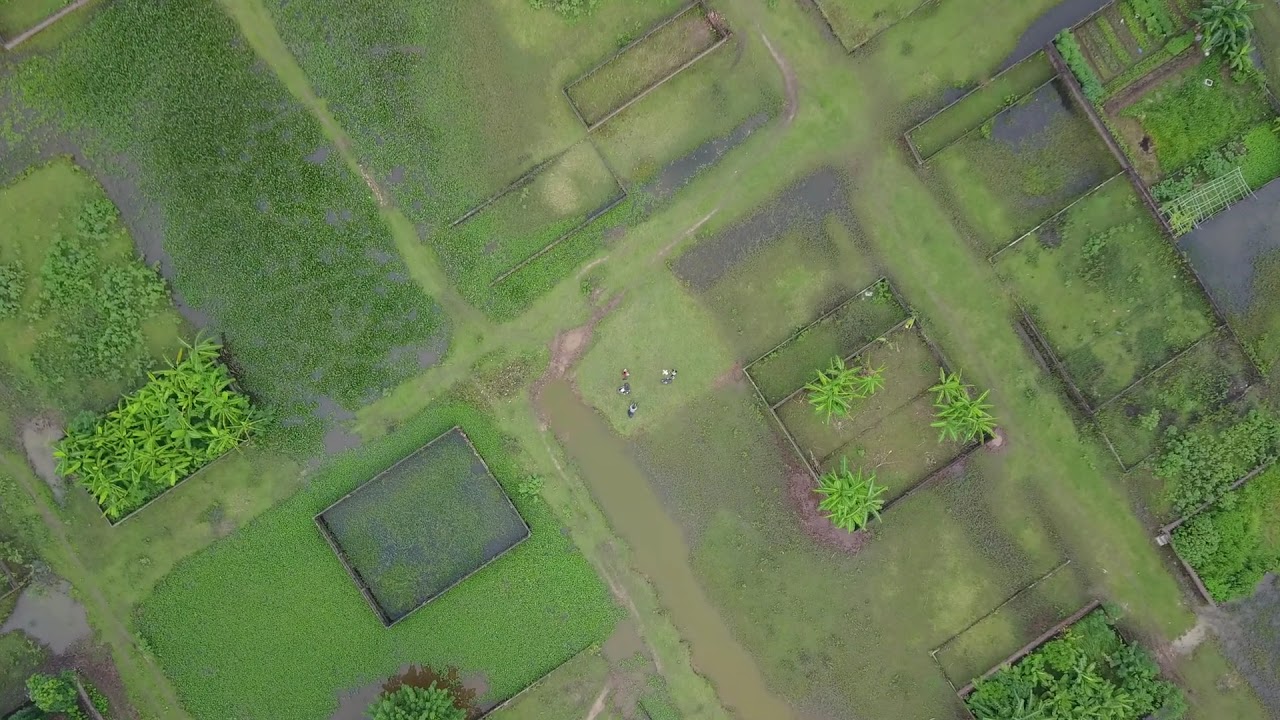An aerial shot reveals a large, horizontally oriented rectangular area divided into multiple sections of varying shades of green, with a few lighter and darker patches interspersed. The landscape is predominantly a bright green, suggesting a healthy, grassy field or farm. Here and there, some sections appear bare, showing gray or light brown earth beneath, with hints of moss. Certain areas contain rectangular enclosures, some of which house light green plants resembling small palm branches, while others are empty. The growing plants appear to be more vibrant in the middle left and left side of the image. Towards the center, and slightly off-center, the sections contain darker green vegetation, possibly denser plants or crops, although the exact nature isn't clear due to the high viewpoint.

In the lower left-hand corner, a large green rectangle envelops a smaller black rectangle, contrasting with its surroundings. Various gray areas appear, particularly in the upper left and upper right sections of the image. Additionally, a strip of brown, which resembles a narrow roadway, extends from the bottom center upwards, cutting through the middle of the field. Scattered roughly at the center of the scene, there are four or five small figures—presumably people—visible but indistinct because of the elevated vantage point.